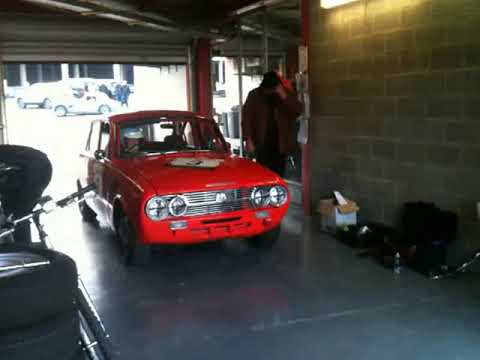The photograph captures a dimly lit garage scene with brick walls and a gray floor. At the center of the image is a small, vintage red sports car, resembling a Mini Cooper from the 60s or 70s, adorned with the number 9 on its side. The car features a shiny exterior, two-round headlights, and a silver grille. A person wearing a white helmet is visible behind the wheel, hinting at a racing scenario. Standing to the right of the car is a man in a burgundy or brown jacket over a black shirt and pants, possibly talking on his phone or describing something. The garage interior includes stacks of tires with a bicycle leaning against them on the left side and an open box with various dark-colored materials on the right. The lighting is minimal, provided by a fluorescent light in the top right corner, casting a dim ambiance. Looking outward, one can see cars parked in the sunlight through the garage entrance.